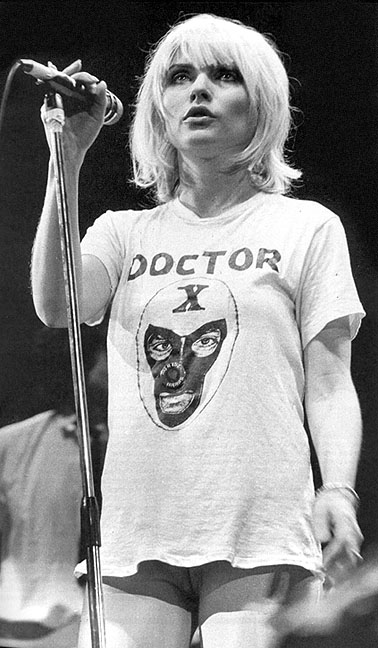In this black and white image, a woman with short blonde hair stands at a microphone attached to a pole. She is wearing a white t-shirt that reads "Dr. X" in black lettering. Below this text is an illustration of a face, seemingly painted black, with a large black X marked on its forehead. The woman's t-shirt is quite long, but it does not fully cover her lower region, revealing her vagina and creating an extremely revealing appearance. Her left wrist is adorned with either a watch or a bracelet. The background is predominantly black, though the blurred presence of another figure, possibly a guitar player, can be discerned. The woman's lips are slightly parted as if she is about to speak or sing into the microphone she is holding. The style of the photograph gives it a vintage feel, and the woman has minimal makeup, except for a touch of black eye makeup.